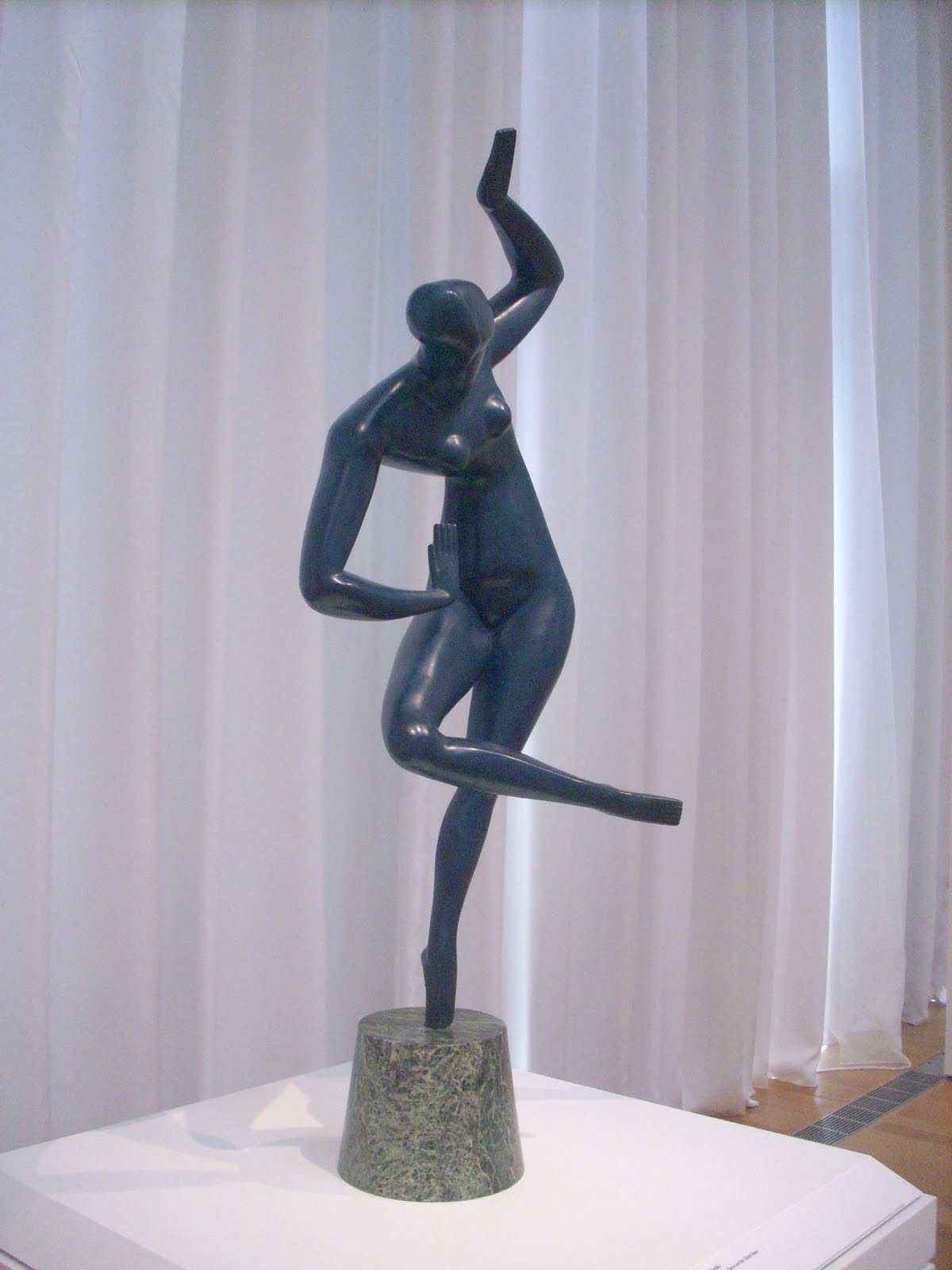This indoor photograph features a detailed sculpture of a woman in a dynamic dancing pose, gracefully balanced on a white cylindrical pedestal. The statue, painted in a deep navy blue, depicts a woman with her left arm flexed and raised above her head while her right arm rests on her waist. One of her legs is bent and lifted, forming a figure-four position, while the toes of her other foot lightly touch the pedestal. The artistic impression includes subtle representations of feminine features, though the head is bent and lacks detailed facial characteristics. Behind the sculpture are white curtains, and a portion of the brown floor, lined with a grey stripe, is visible, suggesting an elegant indoor setting.